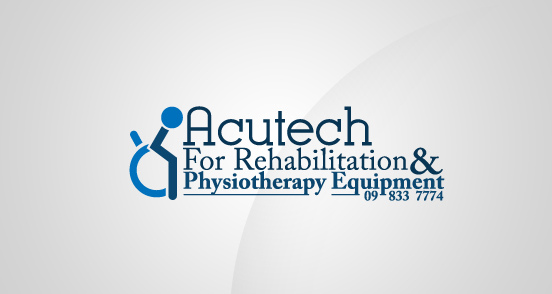The image features the logo and name of a business prominently displayed against a two-toned background. The business is named "AcuTech for Rehabilitation and Physiotherapy Equipment." The logo, positioned to the left of the text, consists of a stylized stick figure in a wheelchair, symbolizing accessibility. This stick figure's head and the wheel are rendered in light blue, while its body is depicted in dark blue. The font used for the business name is dark blue, complementing the logo's colors. Beneath the business name, a phone number, 098337774, is also presented. The background transitions from gray on the right side to off-white on the left side, with a distinct curved line marking the gradient. The overall minimalist design of the image and the central positioning of the text and logo give it a professional appearance, similar to a business card.